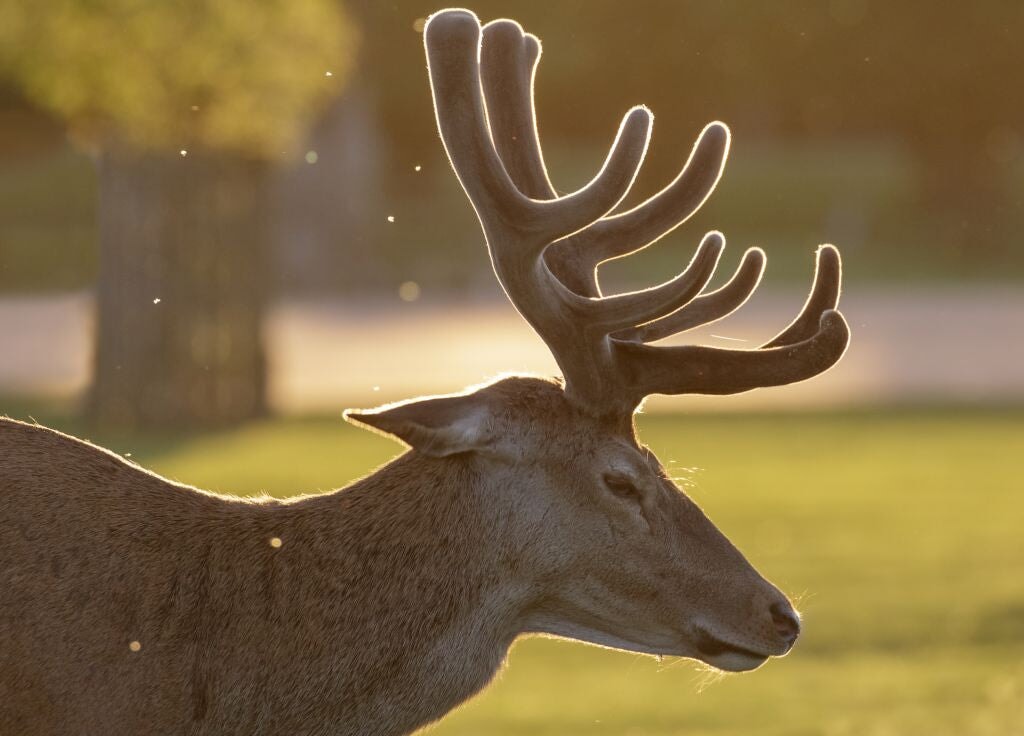This photograph captures a serene outdoor scene featuring a deer, possibly a reindeer, in a rectangular landscape orientation. The deer, positioned coming from the left edge, has its head in the lower center with its nose reaching about three-quarters to the right of the image. Its light brown fur contrasts beautifully with the shiny white outline that highlights not just its body but also its distinct antlers. These antlers emanate majestically from its forehead, with two or three branches extending backwards and other branches, six in total, curling forward in rows of two.

The deer’s ears are slightly down and to the back, adding to its calm and composed demeanor. Its black eyes and nose stand out against the brighter fur, which displays patches of white under its chin and inside the ears. 

In the blurred background, a sunny day is suggested by the bright lighting and the long shadows cast by the deer. A tree trunk with yellowish-green leaves occupies the upper left corner, and there's a suggestion of a road running across the scene. The field of low-cut green grass underlines the deer's tranquil environment. Notably, peculiar light effects and camera aberrations create an almost surreal atmosphere, accentuating the deer’s presence which almost appears to be superimposed against the lush, natural backdrop.